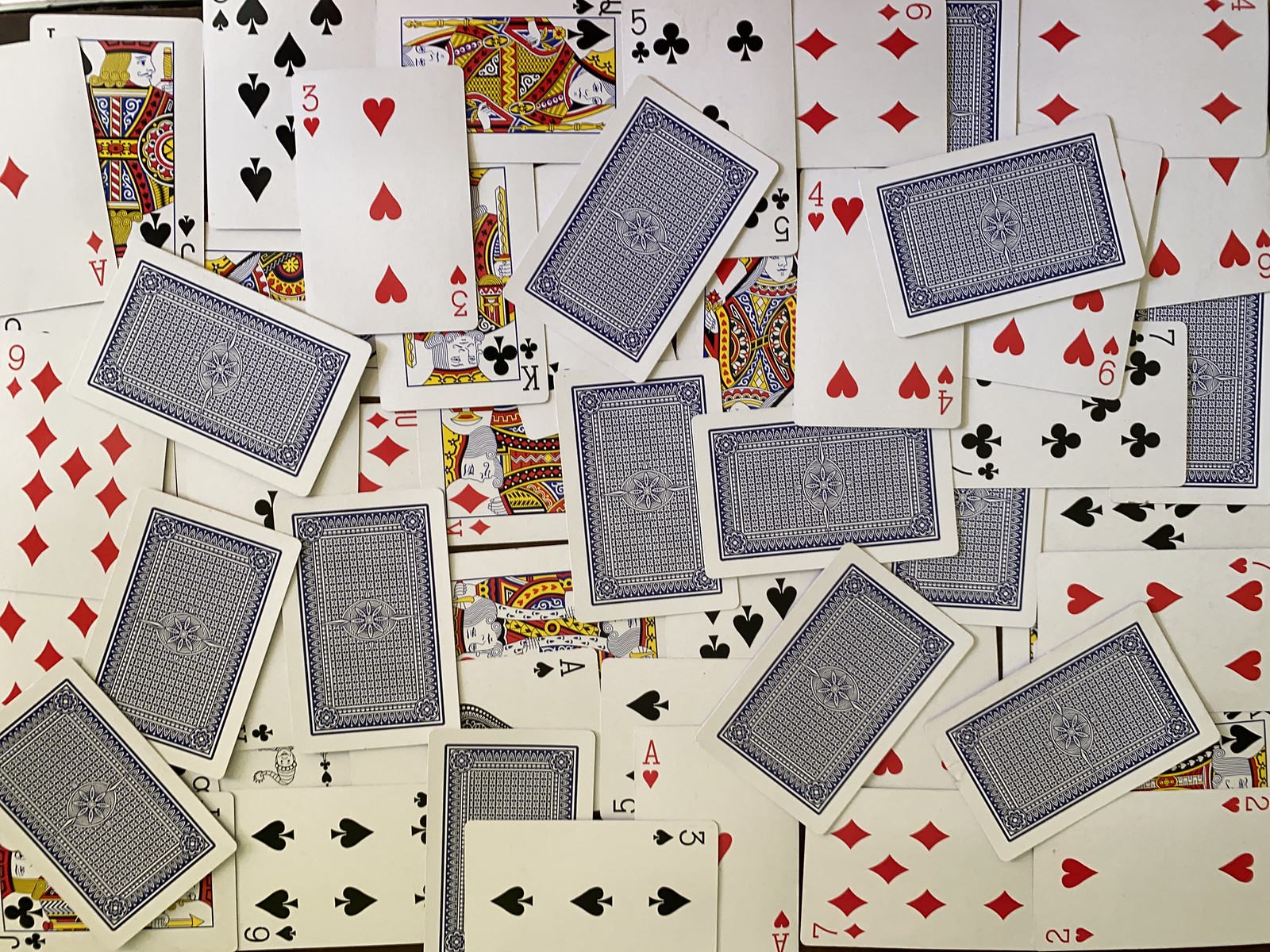A large, scattered pile of playing cards dominates the image, showcasing both face-up and face-down cards. The face-up cards reveal a variety of ranks and suits, including the Ace of Diamonds, 3 of Hearts, Jack of Spades, 9 of Diamonds, 6 of Spades, 3 of Spades, Ace of Hearts, Ace of Spades, 7 of Diamonds, 2 of Hearts, 7 of Hearts, 6 of Hearts, 4 of Hearts, 6 of Diamonds, 5 of Spades, Queen of Spades, King of Clubs, King of Diamonds, 10 of Diamonds, 4 of Diamonds, 6 of Hearts, 2 of Hearts, and King of Spades. The face-down cards, totaling fourteen, have a distinctive back pattern featuring a blue checkered design with a central star or flower motif. The cards overlap and cover one another, creating a rich, textured composition that invites closer inspection.